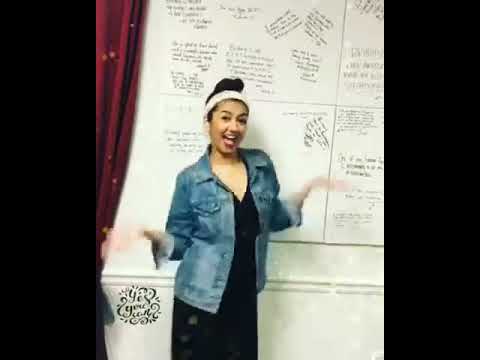In the center of this square-shaped picture, framed by two solid black vertical borders on each side, stands a woman in her mid-30s, smiling broadly with her mouth wide open as if in mid-laugh. She has dark hair, accentuated by a white headband, and is dressed in a denim jacket over a v-neck black dress. Her hands are blurred in motion, extended out to her sides in a "what's happening?" gesture, adding a dynamic element to the image.

The background features a white wall with chair molding at her waist level. Above the molding, there is a whiteboard or similar surface covered with an assortment of text, notes, and messages in various orientations, divided into four sections. To the left of the woman, partially visible, is a burgundy or cranberry-colored curtain, pulled back and adorned with a velvet gold rope. At the bottom left corner of the image, a calligraphy-like design or watermark can be seen, possibly spelling out "yes you can."